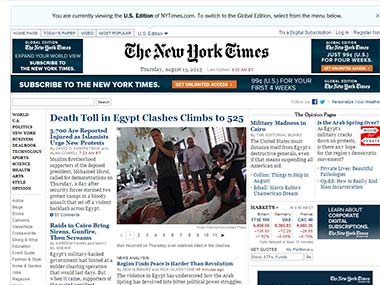The image appears to be a shrunken version of the front page of The New York Times. At the top, the recognizable New York Times logo is flanked by two advertisements. Below the logo is a prominent banner ad promoting a subscription offer: "Subscribe to The New York Times, get unlimited access for just 99 cents USD for your first four weeks," followed by additional, unreadable text.

The main article discusses a significant conflict in Egypt, with the headline: "Death Toll in Egypt Clashes Climbs to 525." Accompanying the article is an impactful photograph showing a distressed man with his hands over his mouth, while another individual appears to be aiding someone on the ground, possibly wounded. The caption beneath the photo mentions that 37,000 people are reported injured, while Islamist groups are calling for new protests.

Below this, there is a series of images highlighting the conflict, with the displayed image being number two out of eleven. Adjacent to the main article is another piece titled "Military Madness in Cairo," containing a brief paragraph and several blue hyperlinks.

The page also includes a section that likely pertains to the stock market, characterized by numerous numbers in red and black, some of which are positive and others negative. Additionally, there are a few more articles with unreadable titles due to the image's reduced size.